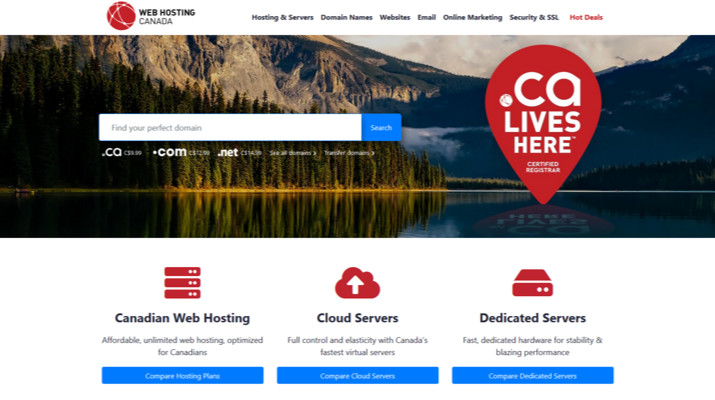A detailed caption for the described image:

"A shot capturing an individual browsing the Web Hosting Canada website. The website's logo is prominently displayed as a circle with four curved lines, creating a spherical appearance. The menu at the top, against a white background, features various options: 'Web Hosting Canada,' 'Hosting and Services,' 'Domain Names,' 'Websites,' 'Email,' 'Online Marketing,' 'Security,' and 'SSL.' On the right side of the menu, a 'Hot Deals' section is indicated.

Below the menu, there's an outdoor image of a serene lake bordered by lush trees climbing a slope, with mountains serving as a picturesque backdrop. The lake, with its placid blue waters, reflects the cloudy sky above. The mountains in the distance showcase green peaks with exposed rocky faces, enhancing the natural beauty of the scene.

The website content highlights various hosting options through clear icons and descriptions. An icon showing server stacks accompanies the text: 'Canadian Web Hosting, affordable unlimited web hosting, optimized for Canadians.' Next is a cloud icon with an arrow, stating: 'Cloud Servers, full control and elasticity with Canada's fastest virtual servers.' Lastly, a server icon introduces 'Dedicated Servers, fast dedicated hardware for stability and blazing performance.'

Underneath these descriptions are light blue buttons with white text, prompting users to 'Compare Hosting Plans,' 'Compare Cloud Services,' and 'Compare Dedicated Servers.'"